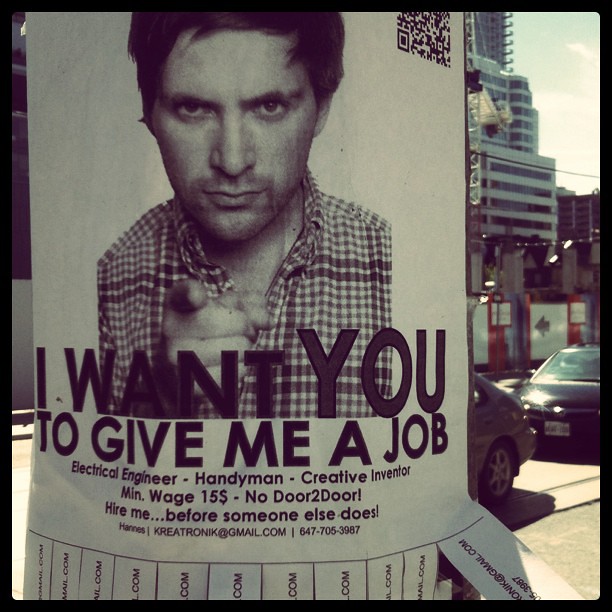This photograph showcases a flyer affixed to a light pole in an urban setting, surrounded by cars and skyline buildings. The centerpiece of the flyer is a black and white image of a stern-looking man pointing directly at the viewer, accompanied by a bold headline that reads, “I want you to give me a job.” Below the headline, the flyer details the man's qualifications, listing electrical engineer, handyman, and creative inventor as his skills, with a minimum acceptable wage of $15 per hour, explicitly stating "no door-to-door" work. The message urges potential employers to “Hire me before someone else does.” At the bottom of the flyer, the contact details are provided as Hannes K-R-E-A-T-R-O-N-I-K at gmail.com and the phone number 647-705-3987. The flyer also features tear-off tabs with the same contact information. The colors of the flyer are muted, predominantly white and gray, blending into the city's backdrop where two cars and modern buildings are discernible.